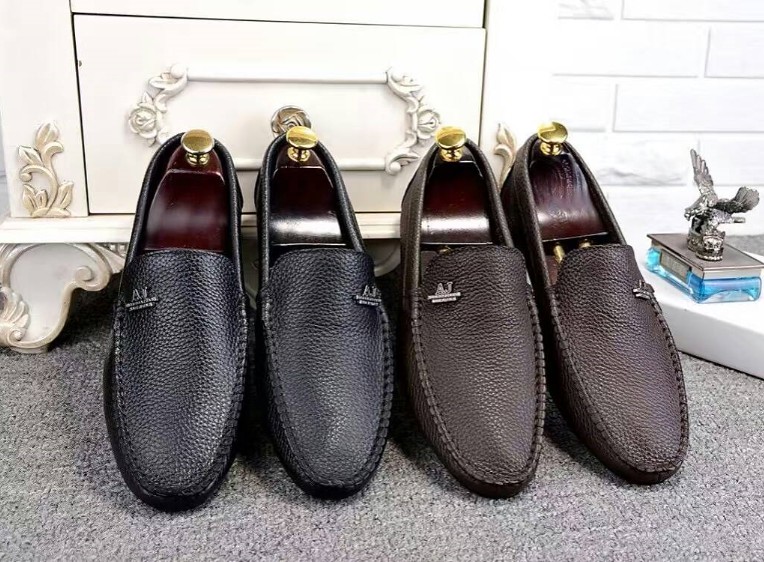The color photograph showcases two pairs of leather loafers resting against a light gray carpet. One pair is black or possibly dark blue, due to the variable lighting, while the other is chocolate brown. Both shoes of the black or dark blue pair come with maroon shoe horns featuring gold handles, whereas the chocolate brown pair also has maroon shoe horns with gold handles. To the right of the shoes, a striking silver eagle statue perched atop a partly silver, partly blue rectangular base is visible. The base, which appears to contain an LCD display and might be an alarm clock, adds an elegant touch. Behind the shoes stands a white drawer adorned with aged, yellowish floral and leaf embroidery. The backdrop includes a brick wall with ornate plaster work, possibly part of a cabinet, adding to the room's intricate detailing. This detailed composition suggests the photograph may have been taken for display purposes, possibly for an online listing or a store's visual merchandising.